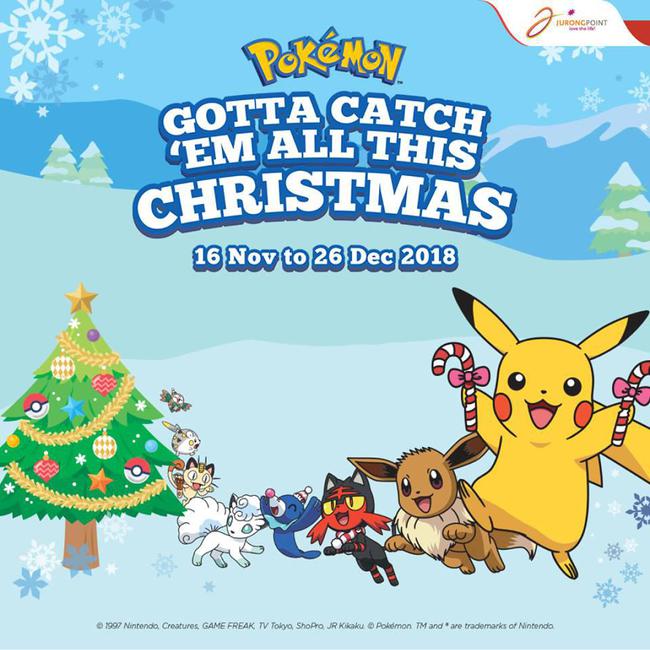A vibrant, festive screenshot featuring a whimsical, blue-tinted cartoon scene adorned with various holiday elements. The backdrop is filled with an array of snowflakes in varying shades, including white, dark blue, light blue, and silver. Dominating the image, a beautifully decorated Christmas tree is festooned with golden garlands and twinkling lights, surrounded by an assortment of animals and candy canes. Among the characters are recognizable Pokémon, interspersed with other anime-styled creatures, all set against a backdrop of snow-covered cartoon trees and mountainous landscapes. The Pokémon logo, prominently displayed in its signature yellow, is accompanied by the catchy phrase, "Gotta catch ‘em all this Christmas." Beneath it, the dates "16 November to 26 December 2018" are listed, emphasizing the promotional event as part of a Nintendo game. At the top of the image is a logo that seems to read "Germ Point," possibly featuring some form of signature or branding, contributing to the overall festive and inviting atmosphere.